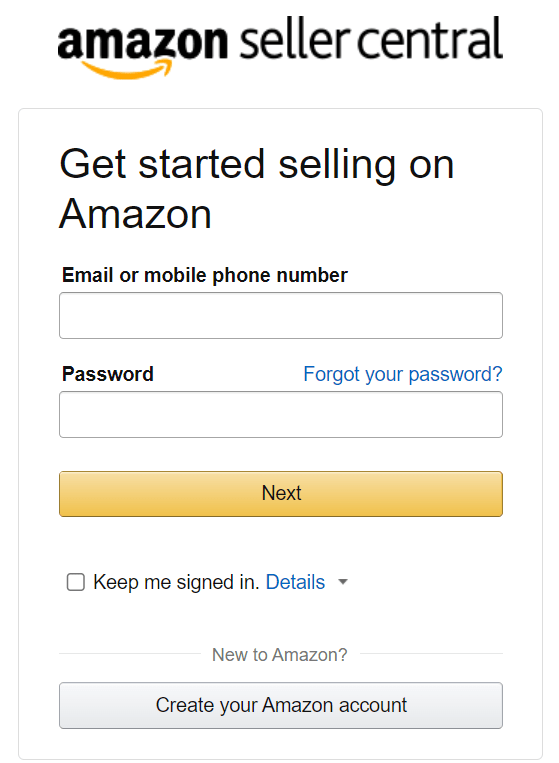The image depicts the Amazon Seller Central login page. At the top center, there is the Amazon logo featuring the iconic yellow arrow. Below the logo, a prominent white box with a gray outline contains the heading "Get started selling on Amazon." Underneath this heading, there is a labeled text box prompting for an "Email or mobile phone number." 

Further below, the page is divided into two sections. The left section is labeled "Password" with an adjacent text box for input, while the right section features a blue hyperlink that reads "Forgot your password?" 

Immediately following, a large yellow rectangular button labeled "Next" is placed centrally. Beneath this button, there is an unchecked box accompanied by the text "Keep me signed in" and a blue hyperlink labeled "Details" with a drop-down menu option beside it.

Towards the bottom of the page, there is a section for new users. It starts with the text "New to Amazon?" positioned above a light gray rectangular box that has a darker gray border. In the center of this box, there is an option that says "Create your Amazon account."